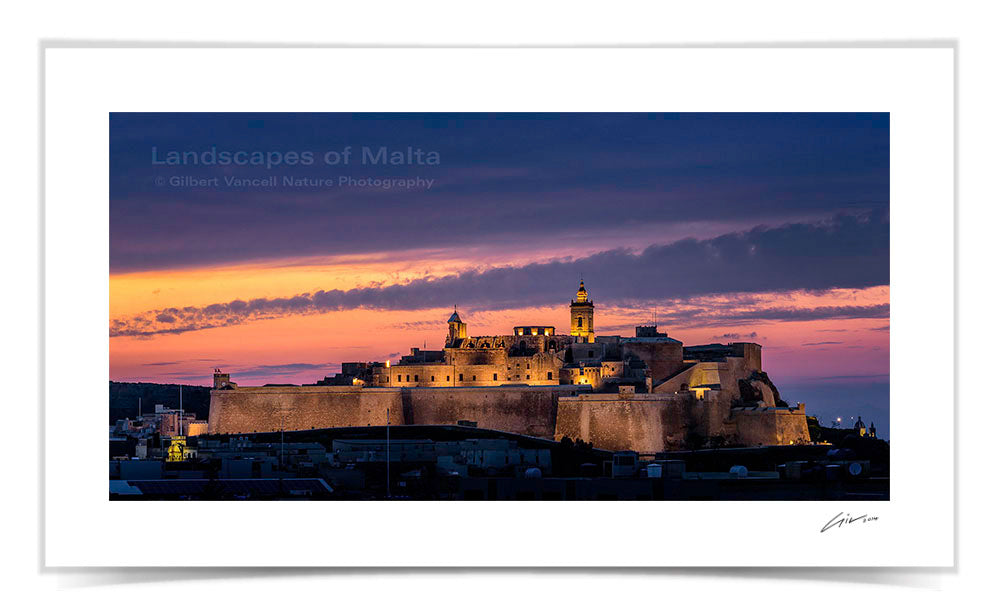This is a detailed photograph with a predominant white border approximately an inch thick, featuring the signature of the photographer, Gilbert Van Coll, in the bottom right-hand corner of the border. The title "Landscapes of Malta" is subtly integrated into the dark, dramatic clouds in the top left-hand corner, along with a label identifying Gilbert Van Coll as a nature photographer.

The image captures a breathtaking sunset, where dark gray and billowing navy blue clouds blend seamlessly into a gradient of rich yellows, pinks, and oranges illuminated by the setting sun. The foreground features a striking, expansive castle-like structure built atop what seems to be a hill or mountain, though the base is shrouded in darkness. 

The castle is surrounded by substantial brown stone walls, with a distinct, illuminated steeple that points sharply into the sky. The structure, appearing fortified and grand, is accentuated by lights that highlight its various features, including several levels of windows and intricate peaks. The overall scene blends the natural beauty of the Maltese landscape with the historic, imposing architecture of the castle, creating a captivating visual narrative.